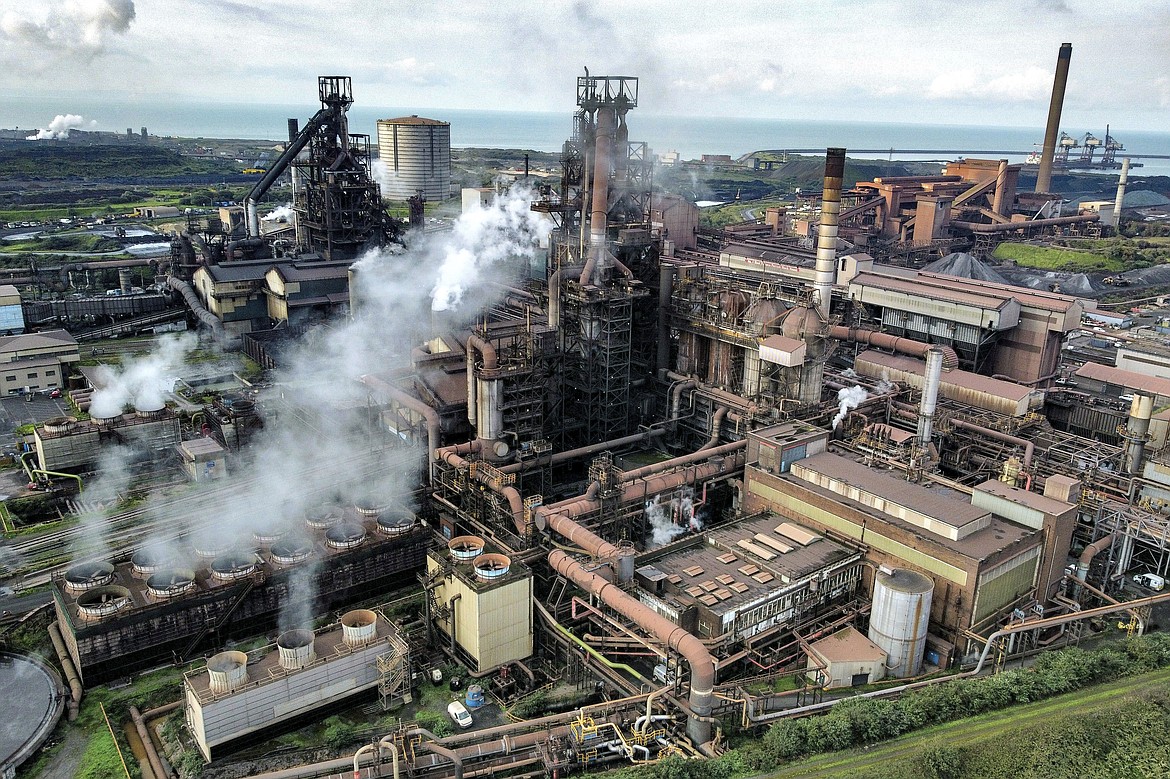This is a highly detailed, professional aerial photograph of a large industrial manufacturing facility, taken on a sunny day, possibly in the morning. The image is oriented horizontally and captures the scene from a few hundred feet in the air, looking slightly downward at an angle. The backdrop features a light blue sky adorned with scattered white clouds and a glimpse of tranquil blue ocean water on the horizon. To the left, the horizon also reveals a small expanse of countryside or a distant cityscape with green grass and scattered buildings.

Dominating the foreground is the sprawling industrial complex with a network of metal buildings, pipes, and exhaust vents. The structures are primarily rectangular and constructed from metal, many of which show signs of age with rust spotting their surfaces. There are tall, dark metal towers emitting white smoke, emphasizing the operational nature of the facility. The complex arrangement of piping and tubing weaves through the buildings, illustrating the intricate functionality of the manufacturing plant. Some rooftops and building sides are visible, tinged with rust-red hues, adding to the aged appearance of the facility.

The bottom of the image is lined with patches of green grass and clusters of green trees, contrasting with the industrial scenery. To the far right, there appears to be a dock or additional industrial section, complete with more materials and structures indicative of the facility's expansive operations. The photograph's sharp focus and extensive detail suggest it may have been professionally taken, possibly for a publication or documentation purpose.